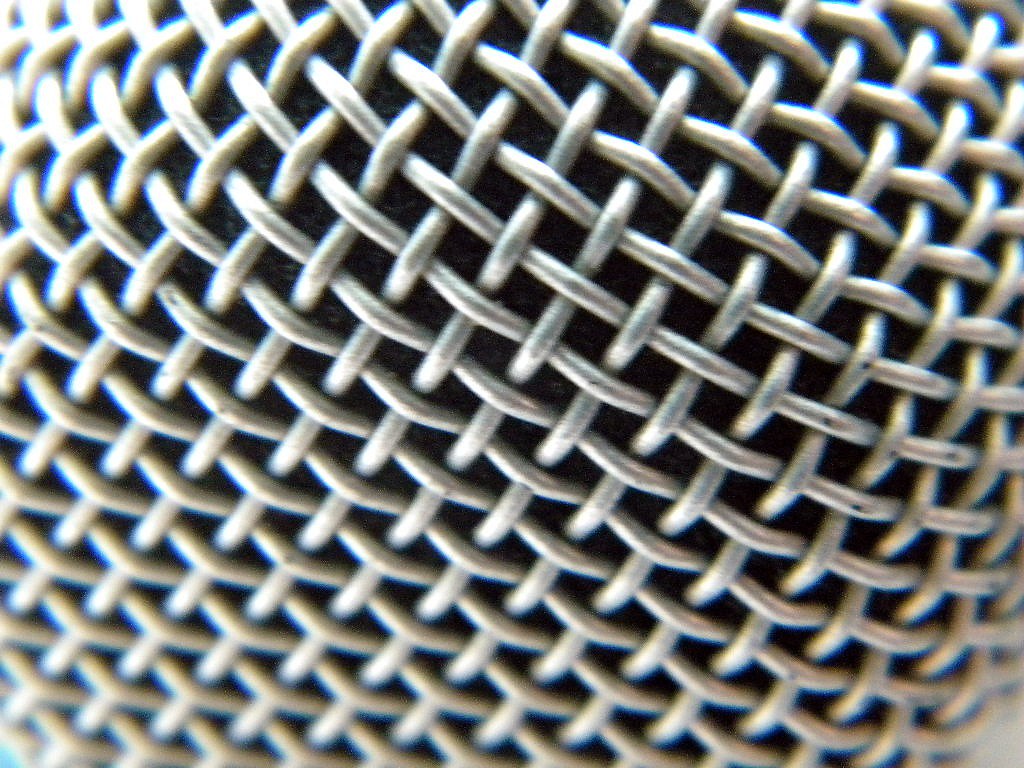The image displays a close-up view of coiled and woven silver metal wires, arranged in a cross-weave pattern, forming multiple small squares. The metal appears heavy and the wires are tightly knit, possibly suggesting a structure resembling a chain or mesh. The center of the image is clearly in focus, showing a bulging round form, indicative of a microphone's mesh or a similar object, while the outer edges, particularly the bottom, are out of focus. The background is a stark black, enhancing the contrast and making the silver wires stand out prominently. Light is coming from the upper left side, casting subtle reflections on the upper portion of the wire coils, which seem to curve back toward the left and the right, possibly hinting at a three-dimensional shape. The detailed weave and reflective quality emphasize the metallic and structured nature of the subject.